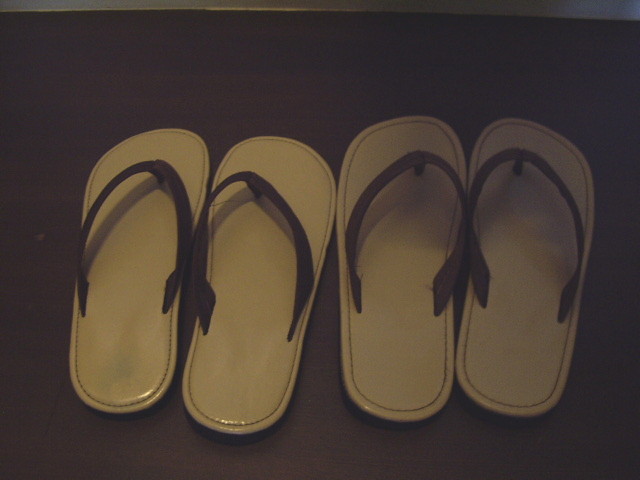This is a slightly out-of-focus, colourised photograph taken from above, depicting two pairs of flip-flop sandals arranged neatly in a row. The sandals feature a light beige or tan base with what appears to be black or dark brown straps that run in a V-shape, going between the big toe and the second toe, and then secured with a central support. The straps and stitching around the sole also appear dark, possibly black. The flip-flops, which are almost rectangular in shape, are placed on a dark brown floor, adding contrast to the scene. In the background, the upper portion of the image transitions from blue on the left to a lighter cream in the center, then darkens back to a near-black before ending in a lighter purple on the right. A reflective light spot can be seen at the bottom edge of the sole on the two left flip-flops. Additionally, a small, bright ray of light is hitting the darker background at the top edge, particularly prominent in the center-right.